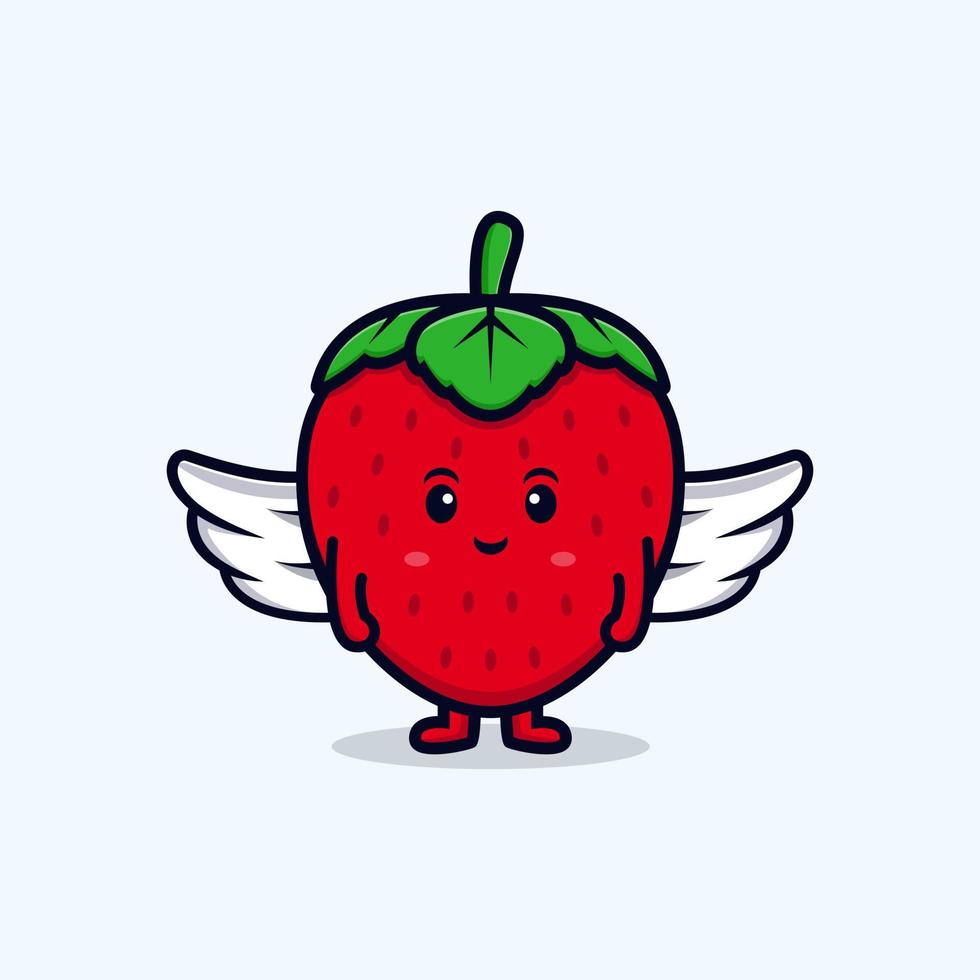This whimsical cartoon illustration features an anthropomorphized bright red strawberry character, centered against a light gray or white background. The strawberry sports a joyful, happy expression with black beady eyes, a black mouth, and pink circular blush marks on its cheeks. Dotting the strawberry's flesh are gray ovals representing seeds. On top, it has a green stem with leaves. The character's arms and legs are depicted as stubby and fingerless, with hands balled into fists. Adding a fantastical element, a pair of white angel wings extend from its back. The strawberry stands on a gray circular shadow, giving the scene a playful and vibrant feel. This character, outlined with thick lines, embodies a cute, fun, and colorful aesthetic, suggesting it might be a prototype for a playful fictional entity or graphic design project.